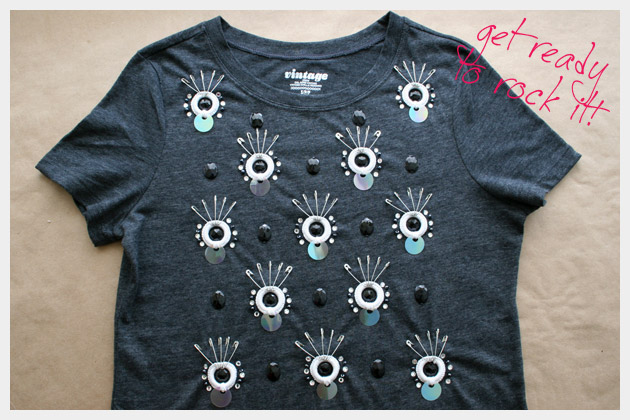The image features a gray short-sleeved shirt that is laying flat on a gray carpet. The shirt, though slightly cut off at the bottom, is the primary focus of the photograph. On the top right corner of the image, there is a playful, scribbly red text that reads, "Get ready to rock it!" followed by an exclamation point. The shirt itself is adorned with round circular designs, each topped with what appear to be pins, adding a unique and edgy flair to the garment. The detailed texture of both the shirt and the carpet creates an intriguing contrast, making the shirt's design stand out prominently against the neutral background.